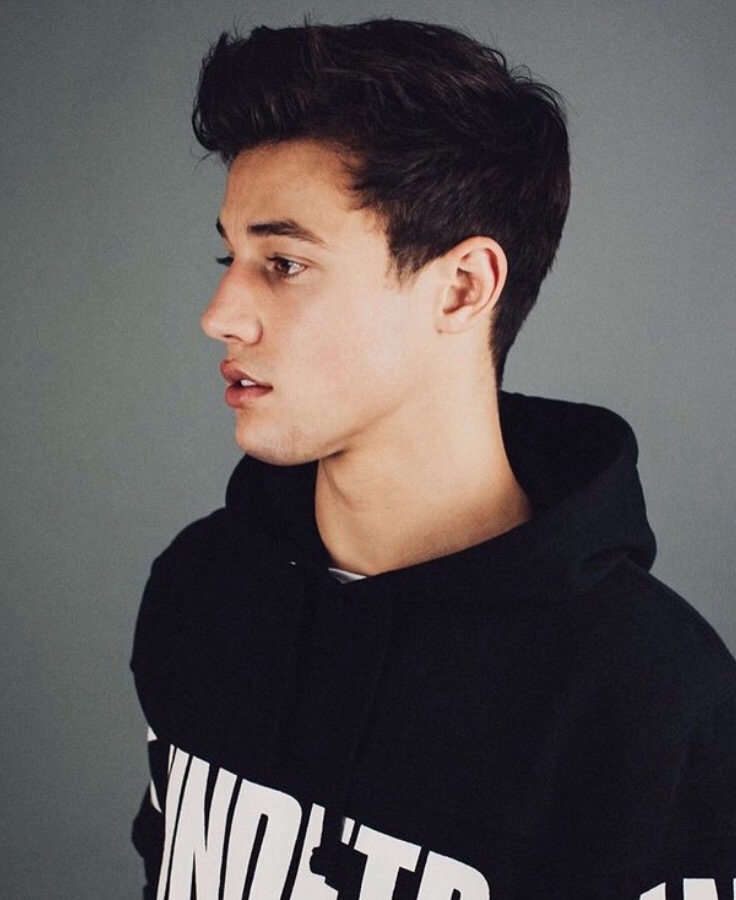The photograph is a color portrait of a young white male with a well-groomed appearance, possibly in his late teens or early 20s. Displayed in a profile view, he faces to the left, allowing us to see the left side of his face. His short, dark brown hair is neatly cut, and he has distinctive brown eyebrows. He possesses a slim neck with a visible Adam's apple. His nose is well-shaped, and his lips have a somewhat deep pink hue, unusual for a boy but perhaps enhanced for the photograph.

The young man is dressed in a black hoodie featuring bold white text, though the visible letters "I, N, A, and D" and parts of "N and T" do not reveal the full wording. Adding to the hoodie’s design, it has white stripes around the sleeves. The backdrop is a gradient gray, lighter in the center and darker around the edges, giving the portrait a studio-like quality. The photo, likely a standard 5x7 inch size, might be something you’d frame, possibly taken for a high school portrait. His light skin, youthful appearance, and neat attire contribute to a clean and composed profile shot.